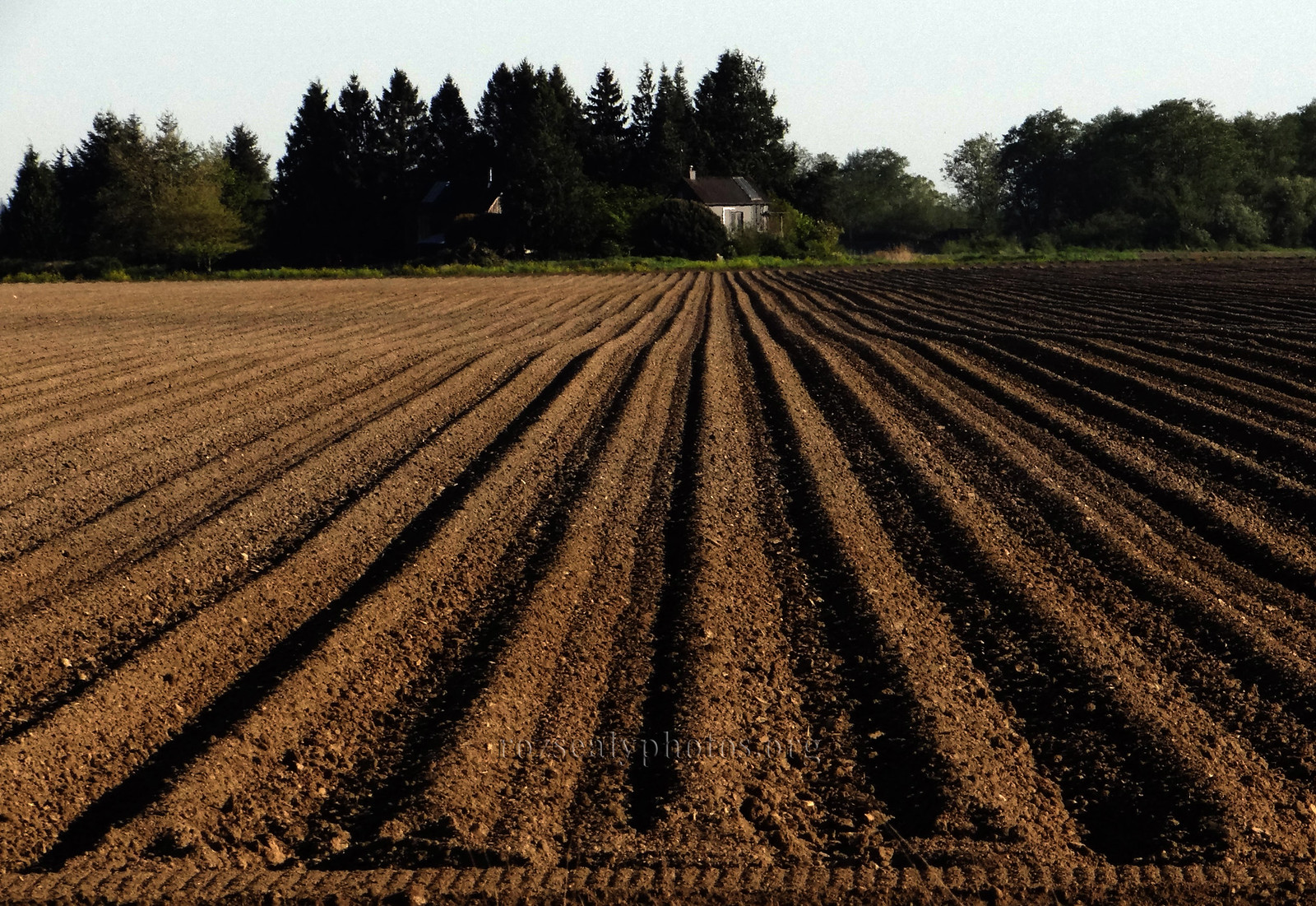The photograph captures a freshly plowed field with perfectly aligned, uniform rows stretching across the expansive plot. The soil is a deep, rich brown, arranged in evenly spaced lines, likely produced by a large machine. The neat rows dominate the lower half of the image, highlighting the preparation for planting.

In the background, a white house, partially obscured by tall, healthy trees, stands at the center. The trees vary in shades of green, creating a lush frame around the house. The roof of the house is a dark color, possibly black, but the shadows from the surrounding trees make it difficult to determine its exact shade.

Above the house, the sky appears hazy, with a mix of white and grayish tones, suggesting either a spring or summer day. At the very bottom center of the image, faint white text is visible, reading “eatsplants.org,” though some preceding numbers are indistinct due to the dark soil background.

Overall, the image offers a scenic view of a meticulously prepared field set against a picturesque rural backdrop, emphasizing the order and readiness for a new planting season.